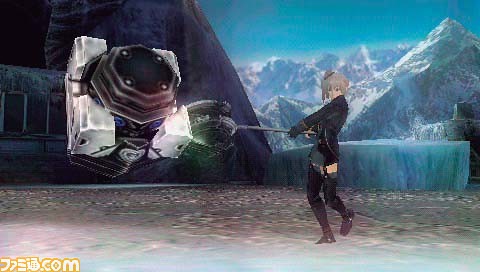In this digitally created landscape-oriented screenshot from a high-tech video game, we see a vividly detailed scene set against a gradient blue sky with snow-capped mountain ranges in the background. The closest mountain is particularly rugged, featuring a metallic structure with brass-colored and white pillar-like components emerging from its side. The foreground depicts a brown concrete ground, adding a touch of realism to the scene. 

The central figure is a female character with short blonde hair, donning a black jacket over a blue top which is pulled together by a garter belt connecting to her black stockings. She is also wearing brown boots. She wields a gray pipe-like staff, which she appears to be swinging while facing the camera. On the bottom left corner of the image, there's a yellow watermark with Japanese characters, possibly including katakana and kanji, followed by “.com,” though it is difficult to decipher fully.